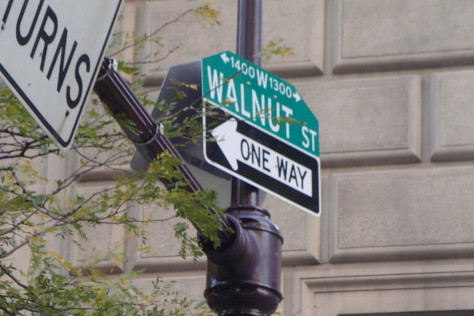This landscape-oriented photograph captures an outdoor scene during the daytime, focusing on a road sign. In the center, mounted on a brown metal pole, is a green street sign that reads "Walnut St." The sign is divided into directional segments, with the letter "W" at the top. Below it, the number "1400" points left, and "1300" points right. Beneath this, a one-way sign with a black arrow directs traffic to the left. A cross arm extends toward the upper left corner of the photo, holding a white sign with black lettering, of which the word "turns" is partially visible in the bottom right corner.

In the background, the façade of a large building, constructed with stone, provides a textured backdrop. Additionally, greenery is visible in the lower left corner, suggesting nearby landscaping. The photo, taken from street level, looks upward at the signage, presenting a clear, detailed view of the street and directional indicators in a bustling urban environment.